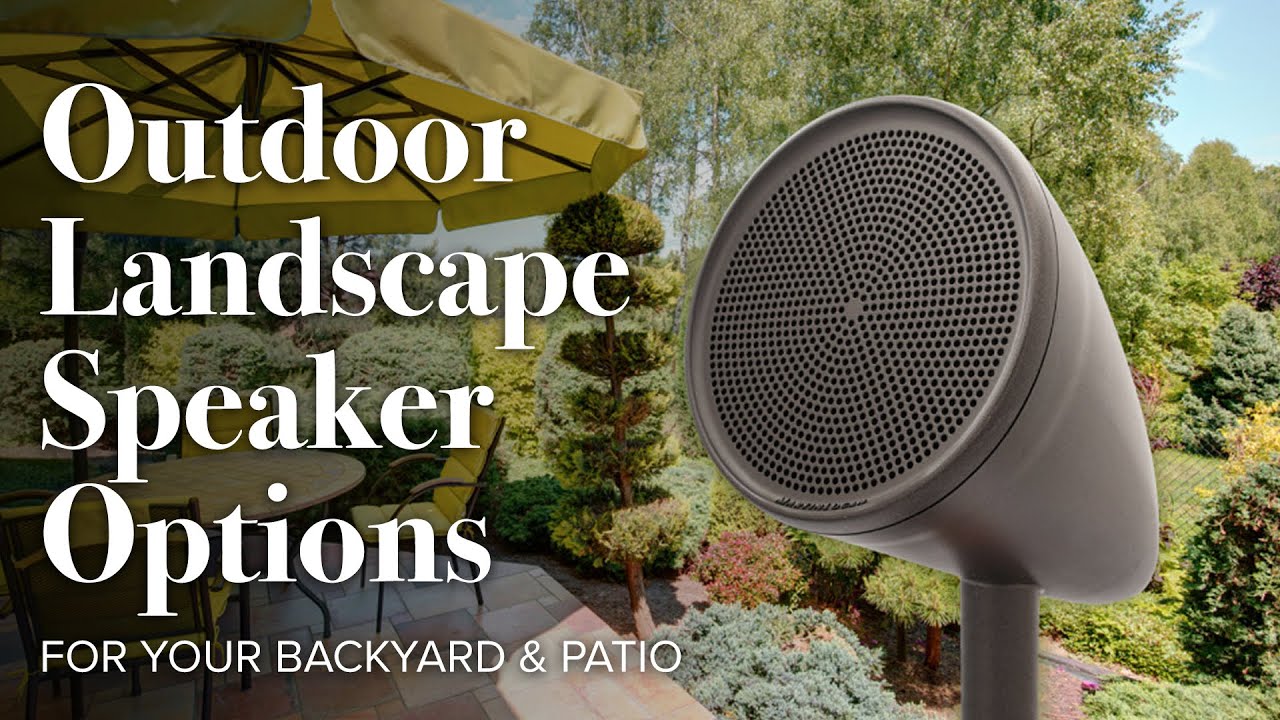This image is an advertisement for outdoor landscape speakers, featuring the text "Outdoor Landscape Speaker Options" in white serif font, and "For Your Backyard and Patio" beneath it in a sand serif, all-caps font. The right side showcases a tall, conical gray speaker affixed to a pole, with its port facing up and slightly left. The left side depicts a serene backyard scene; a patio with a circular table under a yellow umbrella, flanked by two yellow chairs. The patio is bordered by a lush, picturesque garden with various green shrubs, colorful flowers, and towering evergreen trees, set against a beautiful blue sky. The terraced landscape suggests a walkable, inviting space, perfect for enjoying music from the featured outdoor speaker.